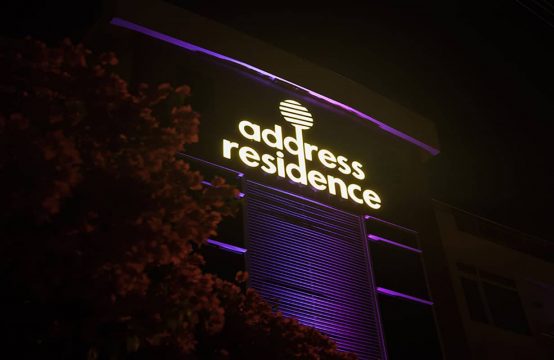The night scene depicts a striking building, likely an apartment or hotel called "Address Residence." The central feature is an illuminated sign with white lettering and a circular logo with black lines, positioned above two front windows. The building is adorned with neon purple lighting, casting a vibrant glow across the roof edge, windows, and middle panel. On the left side of the image, a tree with tightly clumped, red-colored leaves contrasts against the dark, black sky. The building's side wall appears tan with white windows, softly lit by an orange or brown streetlight, possibly a vapor lamp. The dark night sky frames the right side of the image, enhancing the vivid neon illumination of the building.